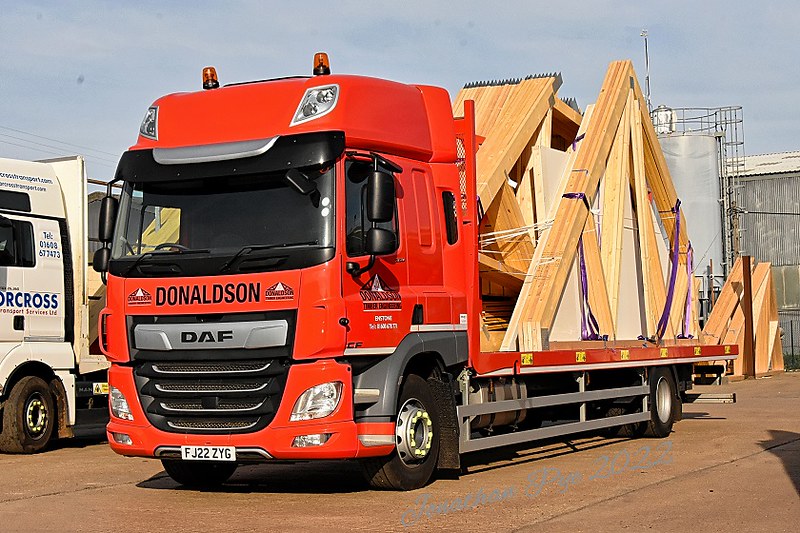The image captures an outdoor setting, likely a construction yard, with a dominant red truck in the foreground. The truck bears the name "Donaldson" prominently in black letters on its front. The front of the truck is equipped with multiple headlights—two on top and four below—and features two small orange lights above the driver and passenger seats. This modern-looking truck has a low flatbed loaded with wooden structures that appear to be prefabricated roof peaks, arranged in triangular formations and securely fastened with purple straps. These wooden structures extend slightly beyond the truck's bed and are tied down carefully. The ground beneath the truck is a brown, wood-like surface, suggesting it is not typical pavement. Adjacent to this red truck is another flatbed truck, white in color. The background includes gray buildings and a ladder, enhancing the impression of a construction environment under a clear, blue sky.